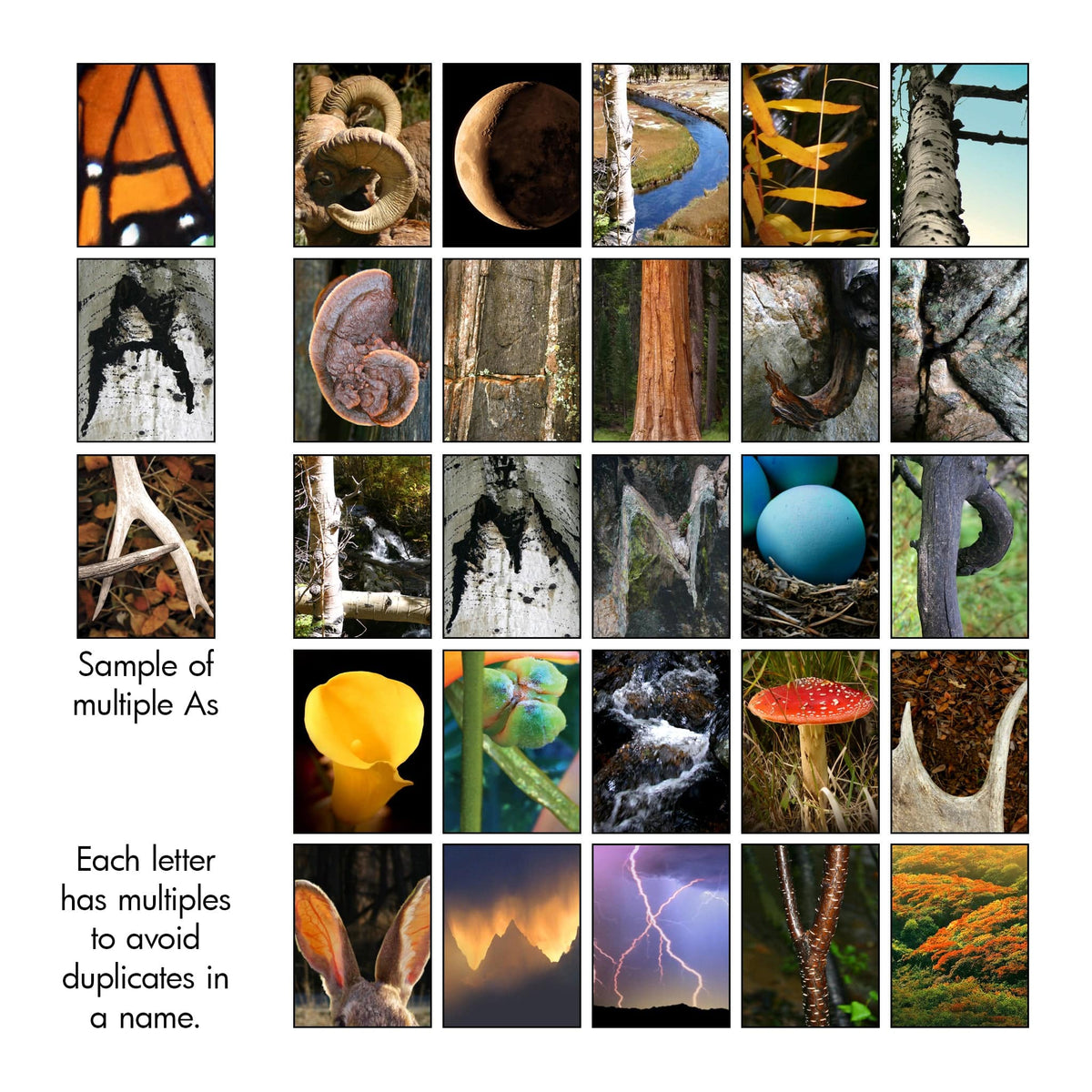This image showcases a series of thirty-three rectangular photographs arranged mostly in a grid with a nature theme. The primary layout on the right consists of 28 images distributed in five rows with the first four rows containing five images each, and the fifth row also having five images. On the left side, a distinct single column contains three photographs, each of the same size and featuring the letter "A" with a caption below them that reads, "Sample of multiple A's, each letter has multiples to avoid duplicates in the name."

In the main grid, each row is filled with detailed nature shots that visually represent different letters of the alphabet:

*Row 1:*
1. A ram's horn
2. A sliver of a crescent moon
3. A shimmering river
4. Green leaves
5. A sturdy birch tree

*Row 2:*
1. Fungi or mushroom on a tree
2. Close-up of a brown tree trunk
3. A crevice in tree bark
4. The letter "K" inscribed in stone

*Row 3:*
1. A white birch tree close-up
2. The letter "M" etched onto a birch tree
3. The letter "N" inscribed on a gray surface
4. Three blue eggs nestled in a nest
5. A weathered gray tree trunk

*Row 4:*
1. A vivid yellow flower close-up
2. A lush green plant close-up
3. A frozen river surrounded by rocks
4. An orange mushroom
5. A close-up of an antler

*Row 5:*
1. Bunny ears
2. Majestic mountains in the background
3. A dramatic electrical storm with lightning
4. A tree branch forming a Y shape
5. A verdant orange and green valley

Each image is colorful and set against a white background, making the vibrant natural elements stand out. The arrangement mimics letters of the alphabet using different aspects of nature, blending art and the natural world harmoniously.